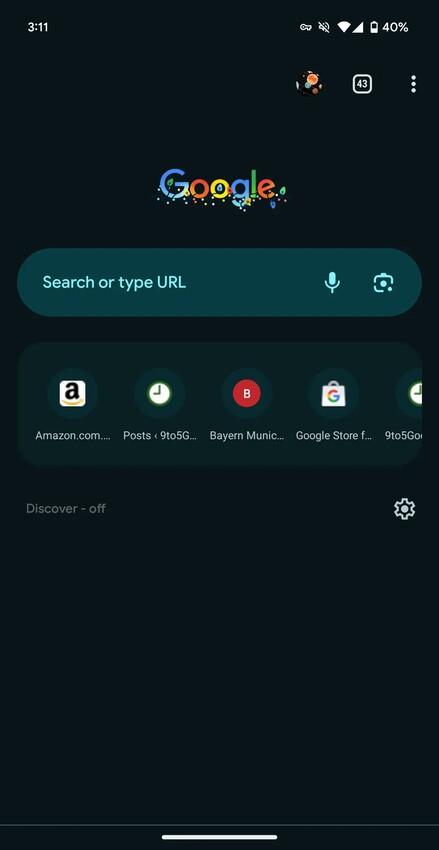The image is of a black page featuring the iconic Google logo in its brightly colored letters at the top. Near the header, there's an unfamiliar symbol resembling a small table tennis paddle angled to the right, surrounded by various colored objects. The screen prominently displays a search bar with the prompt "search or type URL" underneath it. Below this, a series of links are shown: the first one links to Amazon.com, marked by the Amazon logo featuring the characteristic yellow arrow under the black 'A.' The next link, labeled "posts, 9 to 5 gigabytes," is accompanied by a small clock icon. Following that is a red button with a white 'B' in the center, indicating a link to Bayern Munich. Additionally, there's a white briefcase icon with a colorful 'G,' labeled as the Google Store. Another clock icon is visible to the right, followed by a 'Discover' link that is turned off. Finally, there is a settings button.